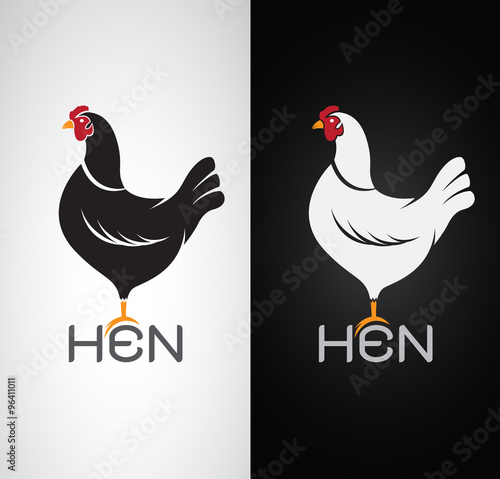This image is a detailed, color illustration presented in a square format divided into two vertical panels, each of equal size. Both panels feature an identical rooster, facing left, depicted in profile. The rooster has distinct red facial features, a gold beak, and a gold clawed foot. Below each rooster is the word "hen," with the rooster's claw touching the curved “E” in the word. The left panel showcases a black rooster against a white background, while the right panel features a white rooster against a black background, creating an inverse color effect. Both panels display a watermark with the text "Adobe Stock" along the left side, indicating it's a digital, purchasable image. The image combines vibrant color illustration with clear typography, emphasizing the contrasting color schemes of the two identical designs.